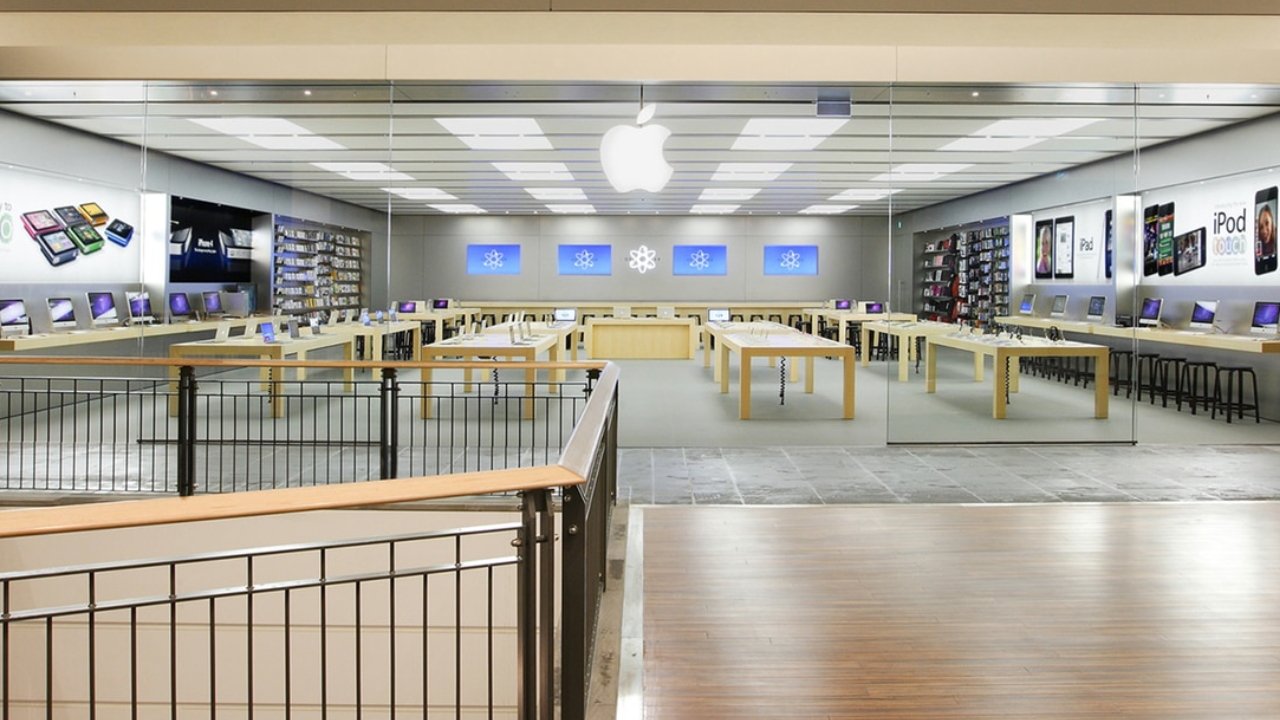The image showcases a bustling Apple Store interior. Upon entering through the six large clear glass panels, two of which are open doors, you are greeted by a sleek, minimalistic design. Central to the store are several desks, arranged in neat rows, each adorned with a dozen laptops available for customer use and examination. Flanking the central area, the walls host additional workstations, each topped with more laptops and interactive displays.

The right side of the store features prominent signage, including an advertisement for iPods, and wall desks accompanied by stools, providing a casual space for customers to explore products. In the back, a series of shelves and racks hold various Apple products and accessories, neatly organized for easy browsing. Above these racks, four screens are mounted on the wall, likely displaying promotional content or helpful information.

At the entrance, an iconic Apple emblem is strategically placed so that opening the doors would split the logo, creating a memorable visual effect. On the left wall, similarly to the right, there are more advertisements for Apple products, additional desks with laptops, and shelves stocked with merchandise.

Overall, the Apple Store exudes a modern, inviting atmosphere with its organized layout of desks, laptops, and product displays, encapsulating the brand's commitment to innovation and customer experience.